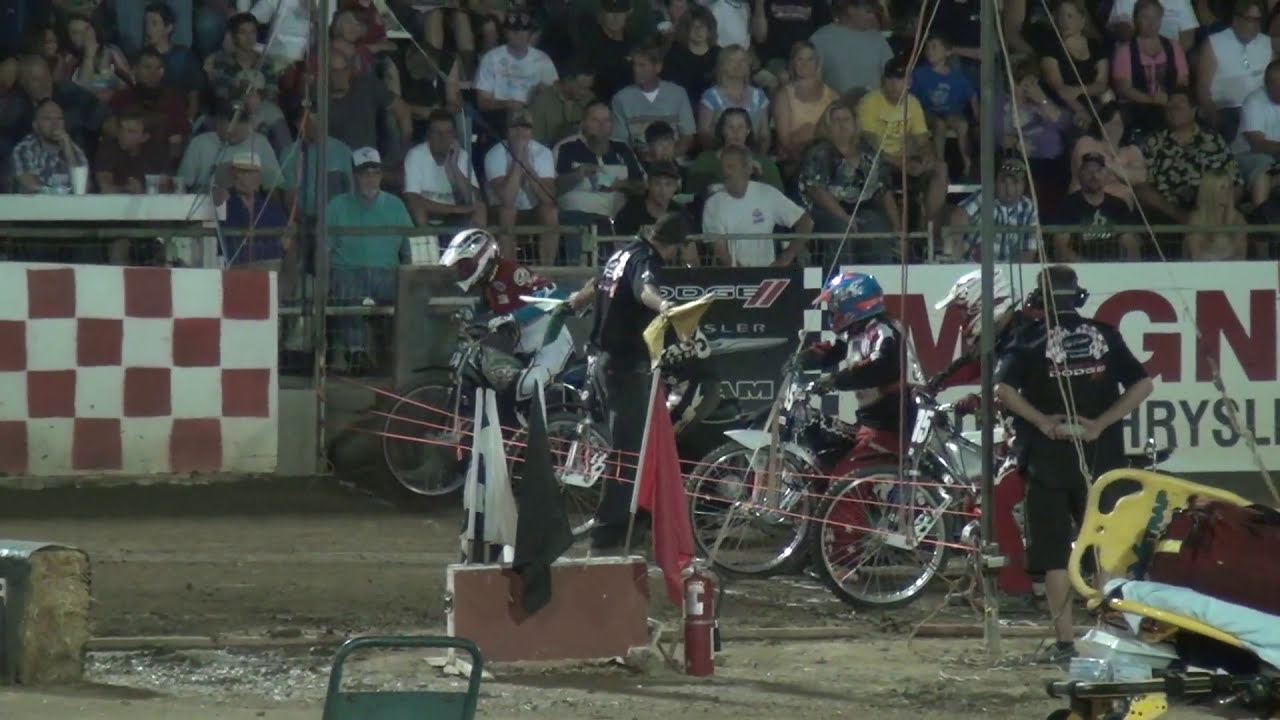This image captures the intense moment at the starting line of a motocross race. In the center of the scene, four motorcyclists are poised on their dirt bikes, wearing helmets and protective gear, aligned against a rope-like starting line on a dirt track. A referee stands at the center with arms extended, holding a yellow and a green flag, signaling the impending start of the race. To the right of the referee is another official, dressed in black with a hat and a headset, possibly for noise protection, standing by the sidelines. Behind the motorcyclists, a vibrant crowd of spectators fills several rows of bleachers, eagerly anticipating the race. The background features a partition wall separating the track from the audience area, adorned with a red and white checkered fence and various advertisements, including a prominent Chrysler sign. On the lower right corner, a gurney is positioned, ready for any potential emergencies. The scene brims with anticipation and excitement as the motorcyclists prepare to launch into the race.